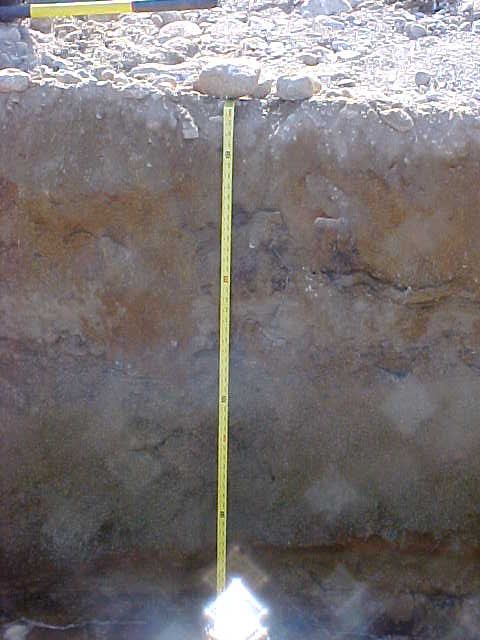The image showcases a rugged rock face, primarily in darker tones with patches of rust and bluish-gray hues. At the very top of the rock formation, a ledge is scattered with numerous white boulders, suggesting recently cleaved or cut nature. A yellow tape measure extends centrally from the top, potentially held in place by stones, descending the cliff face, with discernible black numbering used to measure the height of the cliff. Near the upper left side, a yellow and black tool or padding can be seen, though its exact purpose is unclear due to the angle. Diamond-shaped lights are visible at various points, likely artifact reflections, adding an additional visual layer. The overall impression of the photo suggests an outdoor setting where natural light illuminates the measured geological formation.